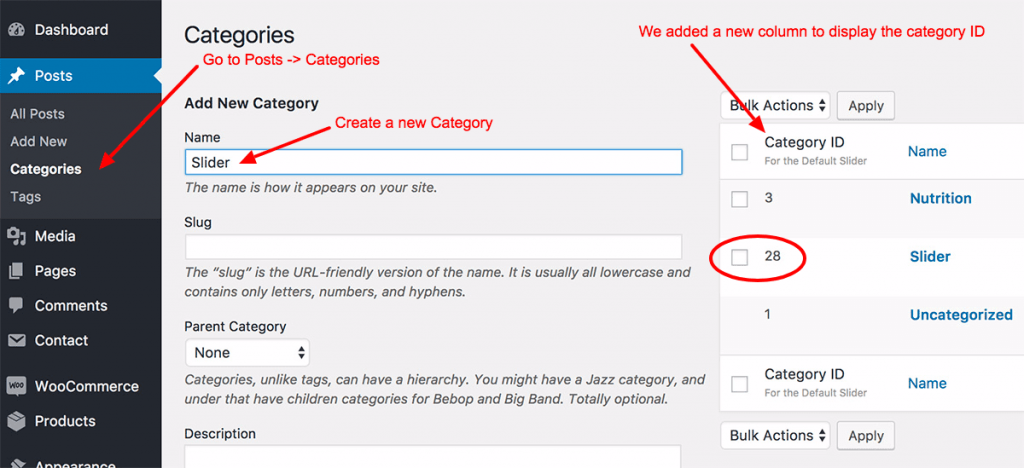The image depicts a customizable dashboard screen with annotations illustrating how to add and manage categories. On the left-hand side, a vertical gray panel lists several options, including 'Posts' and a sub-option 'Categories'. When 'Categories' is selected, the right-hand side of the screen updates to display the category management interface. This interface includes an 'Add New Category' dialog where users can enter the name and properties of a new category.

Several red arrows and text annotations have been superimposed on the screen for clarity. One arrow points to the 'Categories' option under 'Posts', while another indicates where to enter the new category name. Additional arrows highlight the steps to create a new column to display the category ID, with a circle emphasizing the numeric ID of the newly created category. These visual aids guide users through the process of adding and managing categories efficiently.